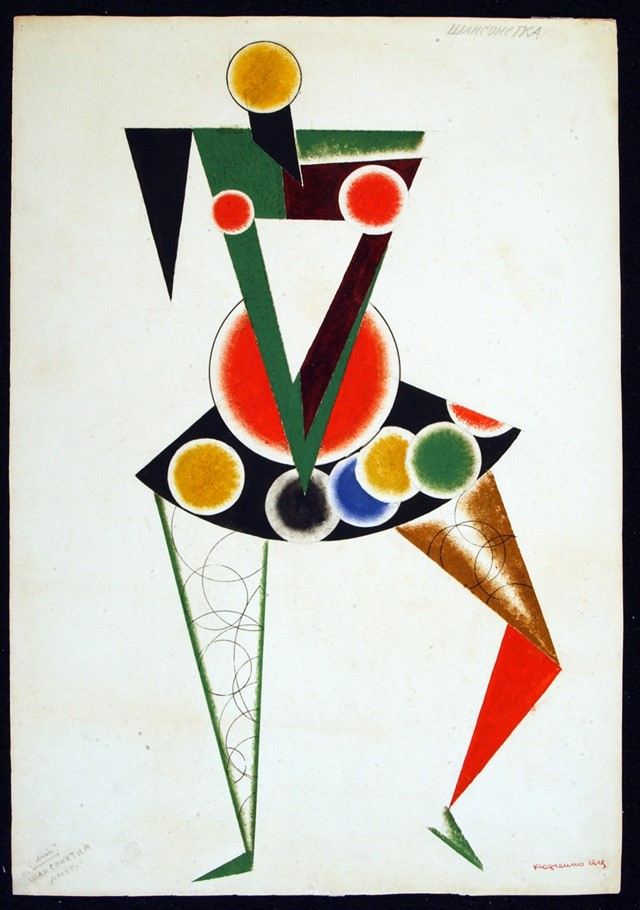This image is a vivid and dynamic abstract painting depicting a stylized human figure, primarily composed of geometric shapes. At the top left portion of the figure, there is a small orangey circle representing the head. Below that, green and black areas suggest shoulders, and two prominent red circles on the chest likely symbolize breasts. The torso tapers into a green and black triangle, reminiscent of the upper body. The skirt of the figure is black and festooned with various colored dots—blue, green, black, and yellow—each trimmed in white, enhancing their distinctiveness. The legs below are fashioned from triangles; the left leg is outlined in green with a white interior, while the right leg features brown, red, and green sections, with subtle swirling details. The background is a light blue, and the entire painting is bordered in black. There is a signature in the bottom left corner and an illegible title on the bottom right, accentuating the artistic nature. This multicolored abstract artwork captures an essence of womanhood without depicting realistic human features, evoking a sense of modern, geometric elegance.